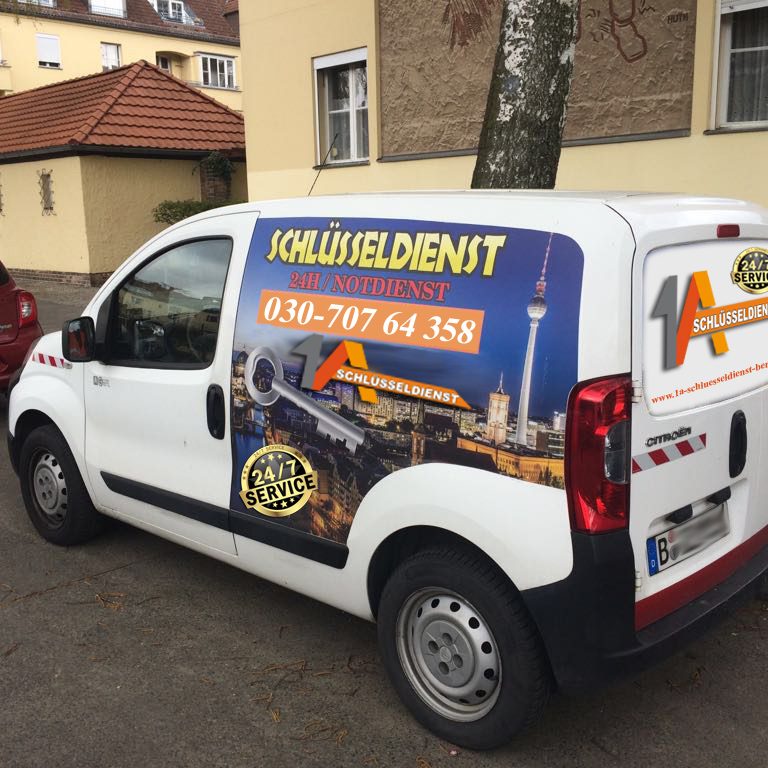The photograph features a white business van, prominently displaying colorful advertisements related to a locksmith service in German. The van is parked on a side street in front of three yellowish buildings and a tree, with another red vehicle partially visible in front of it. The signage on the van includes a large silver key graphic and the words "Schlüsseldienst," indicating it is a locksmith service. The ad is primarily blue with yellow text and highlights a 24-hour service ("24h" and "24-7 service"). Additionally, the phone number "030-707-64358" is displayed within an orange rectangle with white lettering. The key imagery and tall city tower in the background suggest a professional locksmith service that operates around the clock.